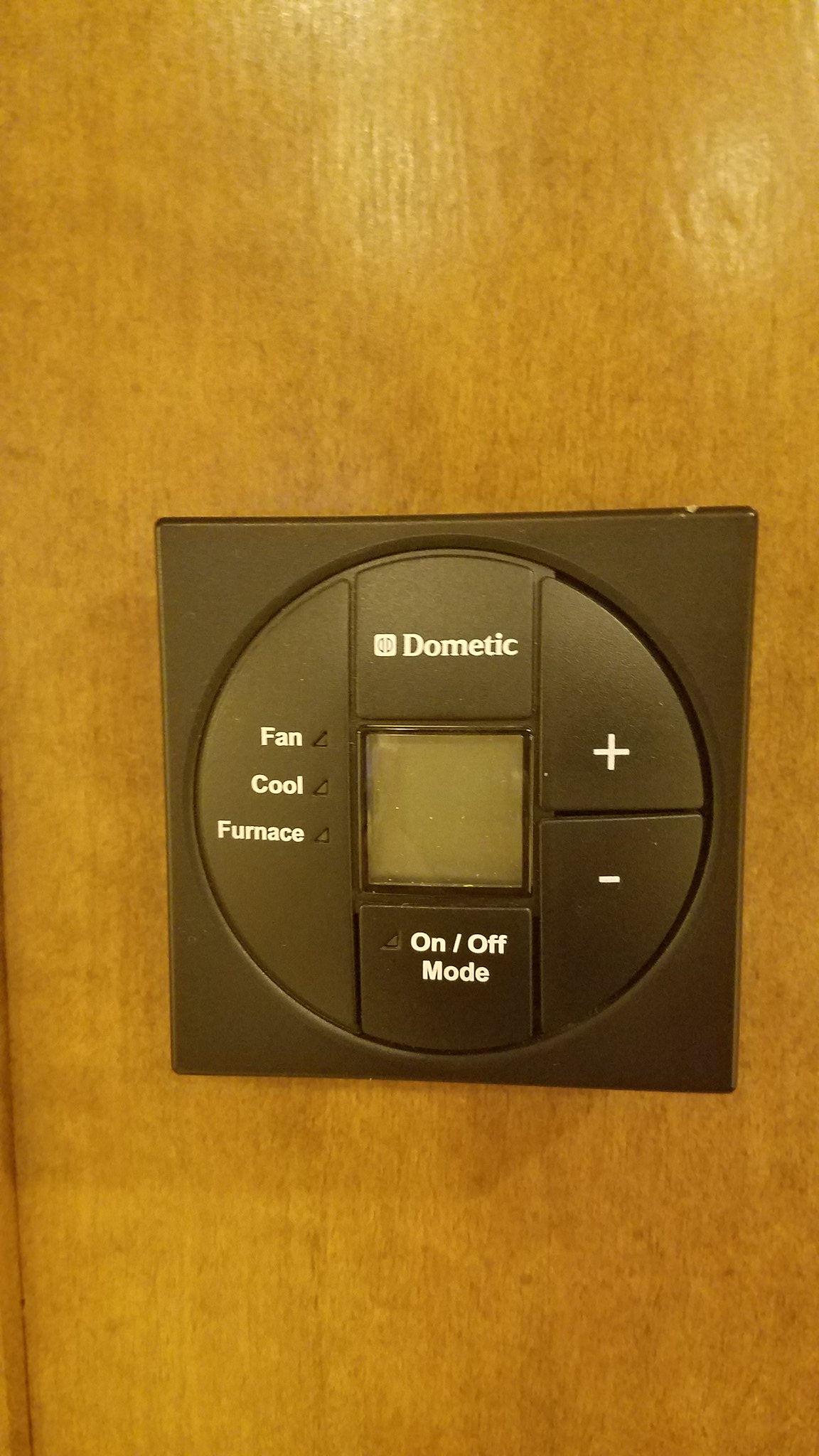A unique thermostat, branded "Dometic," is mounted against a wooden wall, prominently displaying the brand name "Dometic" at the top alongside an indistinct logo. The electronic device features a small viewing window below the brand name, which likely houses the radio control settings. All text on the thermostat is in white. On the left side, labels indicate functions such as "fan," "cool," and "furnace," each accompanied by small indicator lights that presumably signal their active status. The bottom of the unit includes an "on/off mode" label, also with an accompanying light that currently appears to be off. To the right, two semicircular buttons, marked with a plus and minus, likely adjust the temperature. This circular interface resides within a larger square frame that is fixed to the wall. The wall itself is sizable and comprised of light brown-green wood. The thermostat appears to be off, but when activated, it likely displays black text indicating the current temperature, with small gray squares beneath each function name. The left button remains a simple semicircle, while the right is divided into two segments for increasing or decreasing the temperature. The upper section of the device contains small square indicators for "Dometic" and "on/off mode."